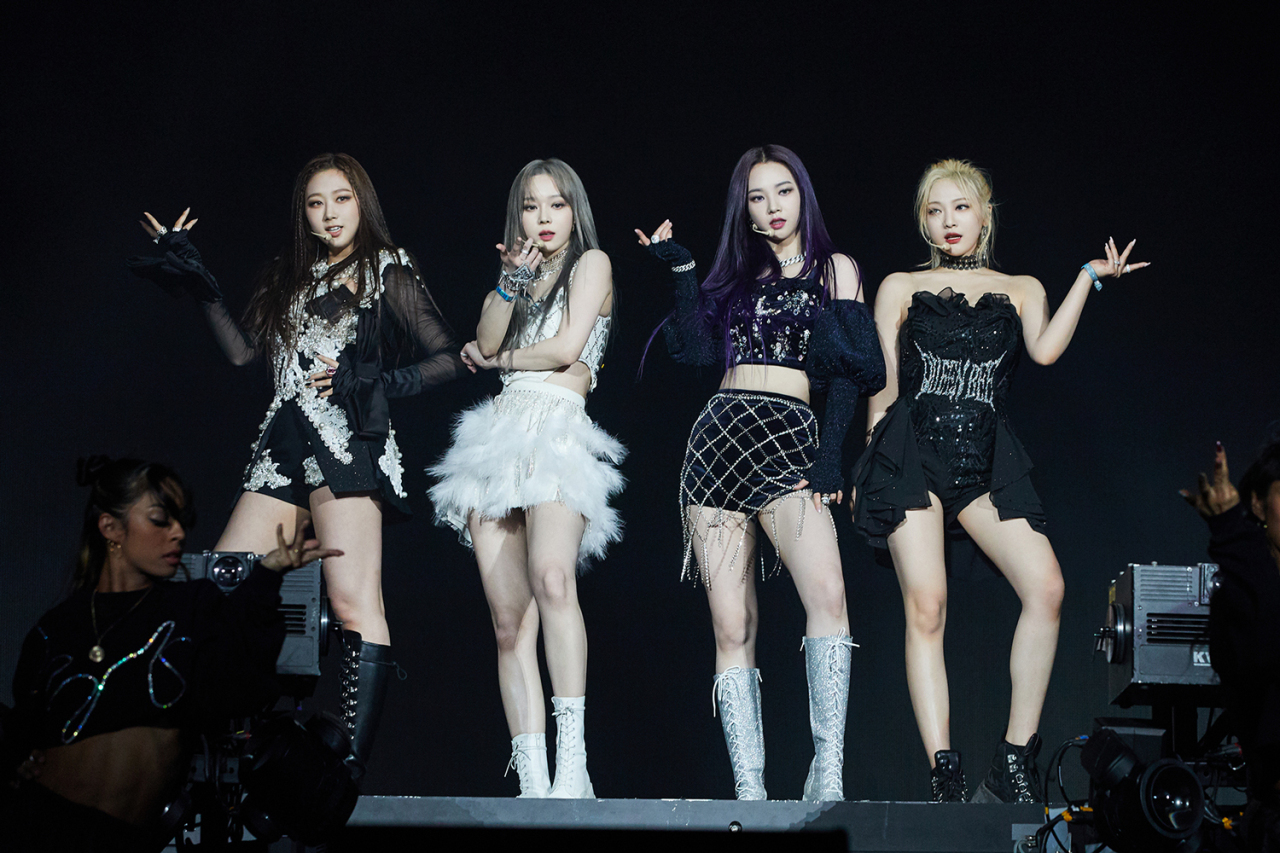This photograph showcases a dynamic performance by a Korean girl band, featuring four members standing prominently at the center of a black stage, under full, focused lighting that enhances their striking appearance. The young woman on the far left is dressed in a black and white dress, complemented by knee-high black boots; her long, loose dark hair and raised right hand with fingers splayed add to her commanding presence. Next to her stands a member in a white dress adorned with corset-style lacing and a fluffy white skirt, her mid-calf length boots gleam under the lights as she appears to blow a kiss towards the audience, her light, loose hair flowing behind her. The third girl from the left stands out in knee-high silver boots and a distinctive black pair of shorts with a chain-skirt overlay, her short top and jacket paired with her raised right hand and intense gaze towards the camera, her dark brown hair adding to her captivating look. On the far right, the fourth member is seen with ankle-high boots, very short shorts detailed with a silver corset, and a small skirt around the back, her blonde hair making a contrast as she directs her left hand towards the audience with her fingers extended. A backup dancer, mostly in shadow but noticeable in the bottom left corner, subtly enhances the scene. The varied yet coordinated stage outfits, featuring blacks, whites, and sparkles, emphasize their unified yet individual styles, while their fair skin and differing hair colors—from dark brown to blonde—add a visual richness to the composition.